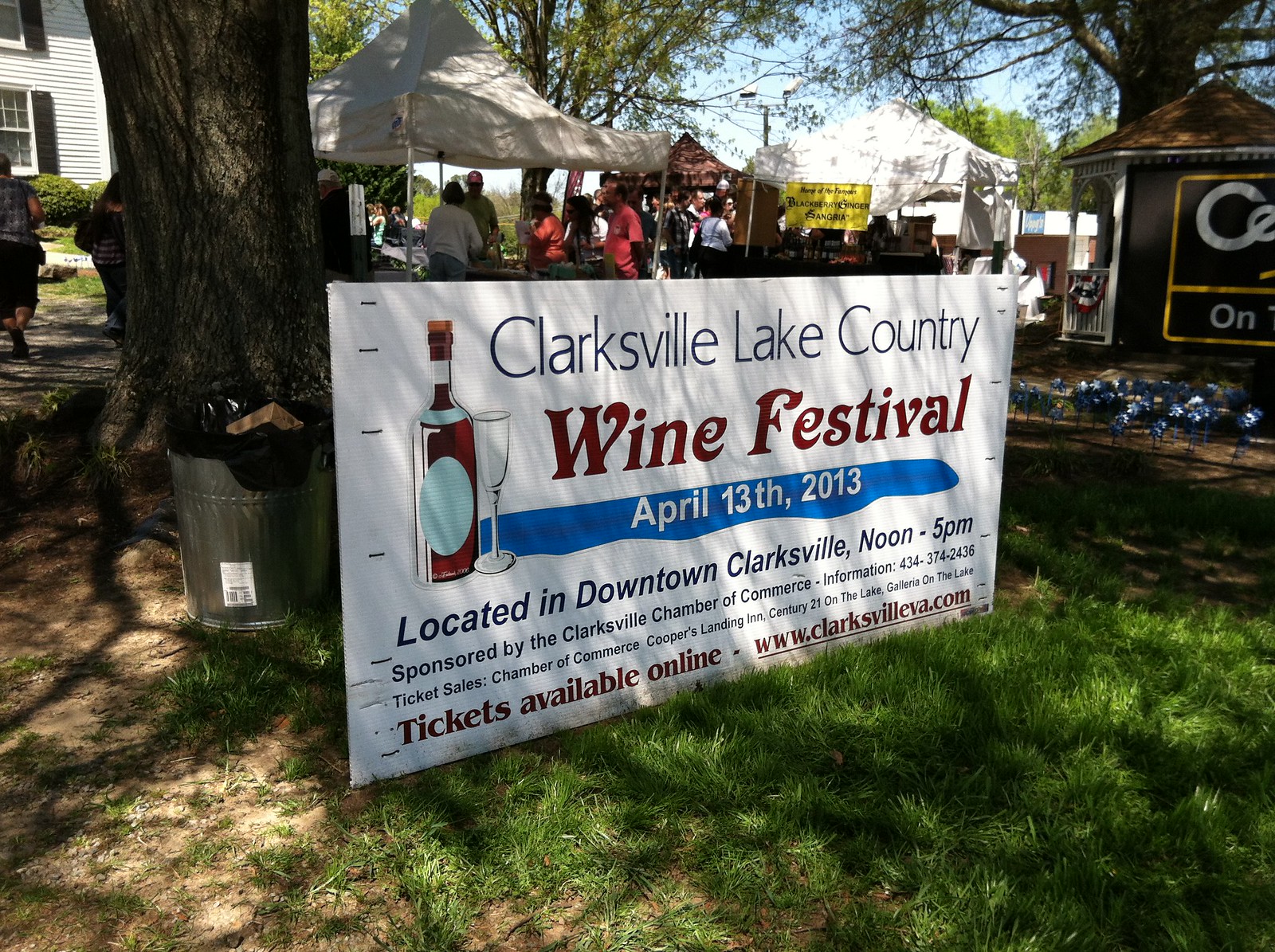The photograph showcases a vibrant outdoor scene featuring a detailed sign for the "Clarksville Lake County Wine Festival" held on April 13, 2013, in downtown Clarksville from noon to 5 PM. The sign, with a white background, is adorned with a cartoon illustration of a wine bottle and glass on its left side. Details in black and brown text include sponsorship by the Clarksville Chamber of Commerce, contact information, and ticket availability at locations such as Cooper’s Landing and Century 21 on the Lake. In the foreground, a metal trash can filled with a protruding brown box stands in front of a lush green tree. Surrounding the central sign, the grass is neatly cut, and a well-maintained park landscape unfolds with white tents hosting numerous attendees. To the right, a charming gazebo with a brown tiled roof displays a large Century 21 sign. The day appears clear and sunny, highlighted by green trees and a bright blue sky, reflecting a lively community gathering.